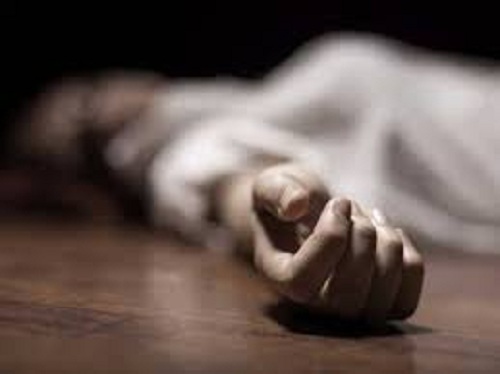This smaller-sized, square picture, devoid of borders, presents a distressingly blurry image of a figure that seems to be female, based on the curvature of the body. The person is lying on their back on a brown wooden or vinyl floor, with their head tilted towards the viewer. The top portion of the picture remains a solid black, providing no backdrop details. The hand in the foreground, identified as the right hand, is stretched out with fingers slightly curled, appearing lifeless and grayish, which adds to the morbid atmosphere of the image. The person is clad in a white top with the sleeves rolled back, though the entirety of their body, especially the face and head, is markedly out of focus. The scene captured is hauntingly ambiguous, suggesting themes of death or severe injury, and could be particularly unsettling for some viewers.